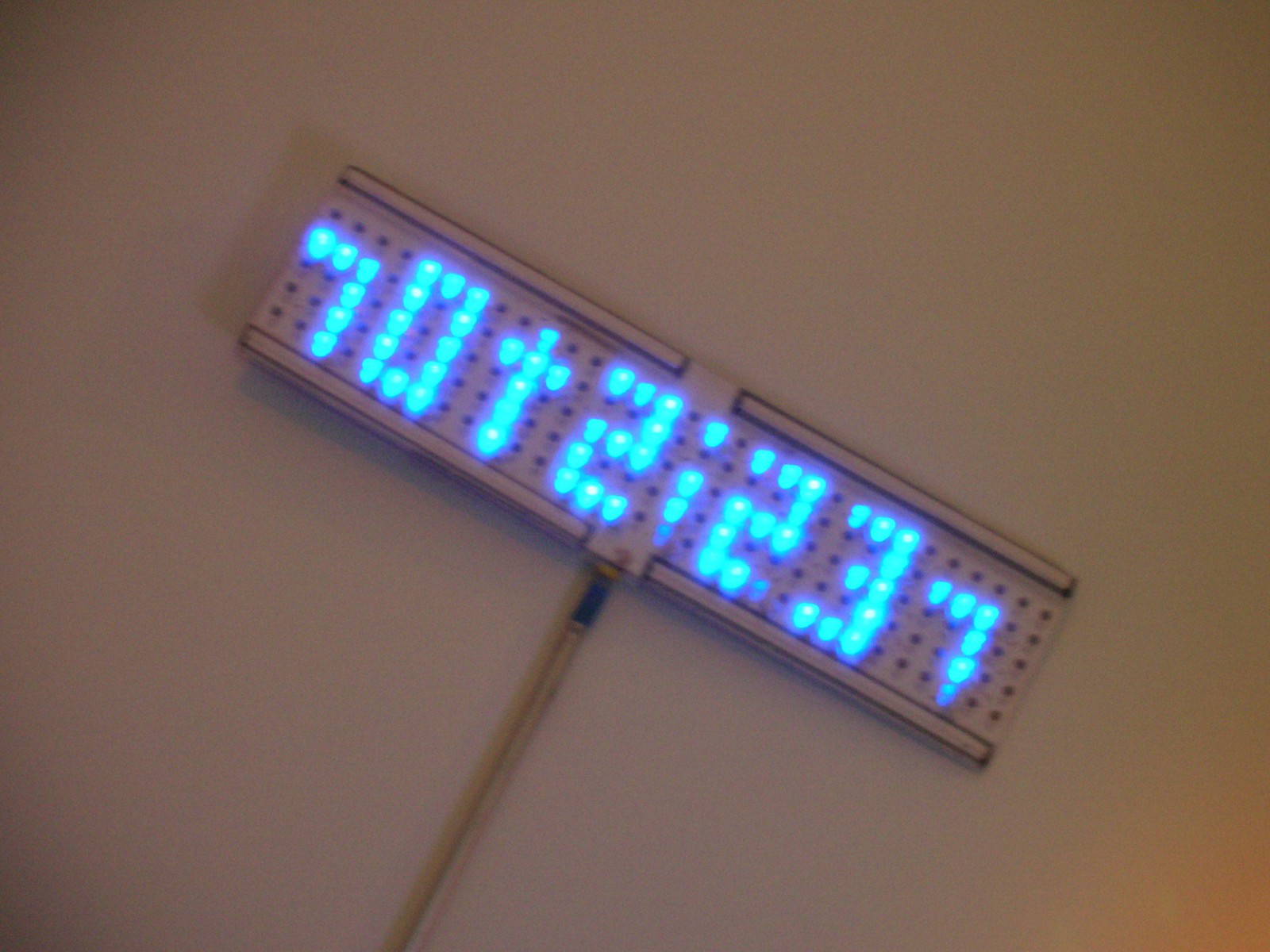In this image, we see an electronic timer affixed to a brown wall, tilted at a 45-degree angle downward to the right. The device features a perforated design similar to a long, skinny cheese grater. Bright baby blue LEDs form the digits "2:23" on this perforated surface. Additional elements include a "7," a "0," and a "+," placed to the left of the time display; however, the smaller-sized "7" may merely be a design feature rather than an actual digit. A post, likely serving as the power source, extends into the timer.